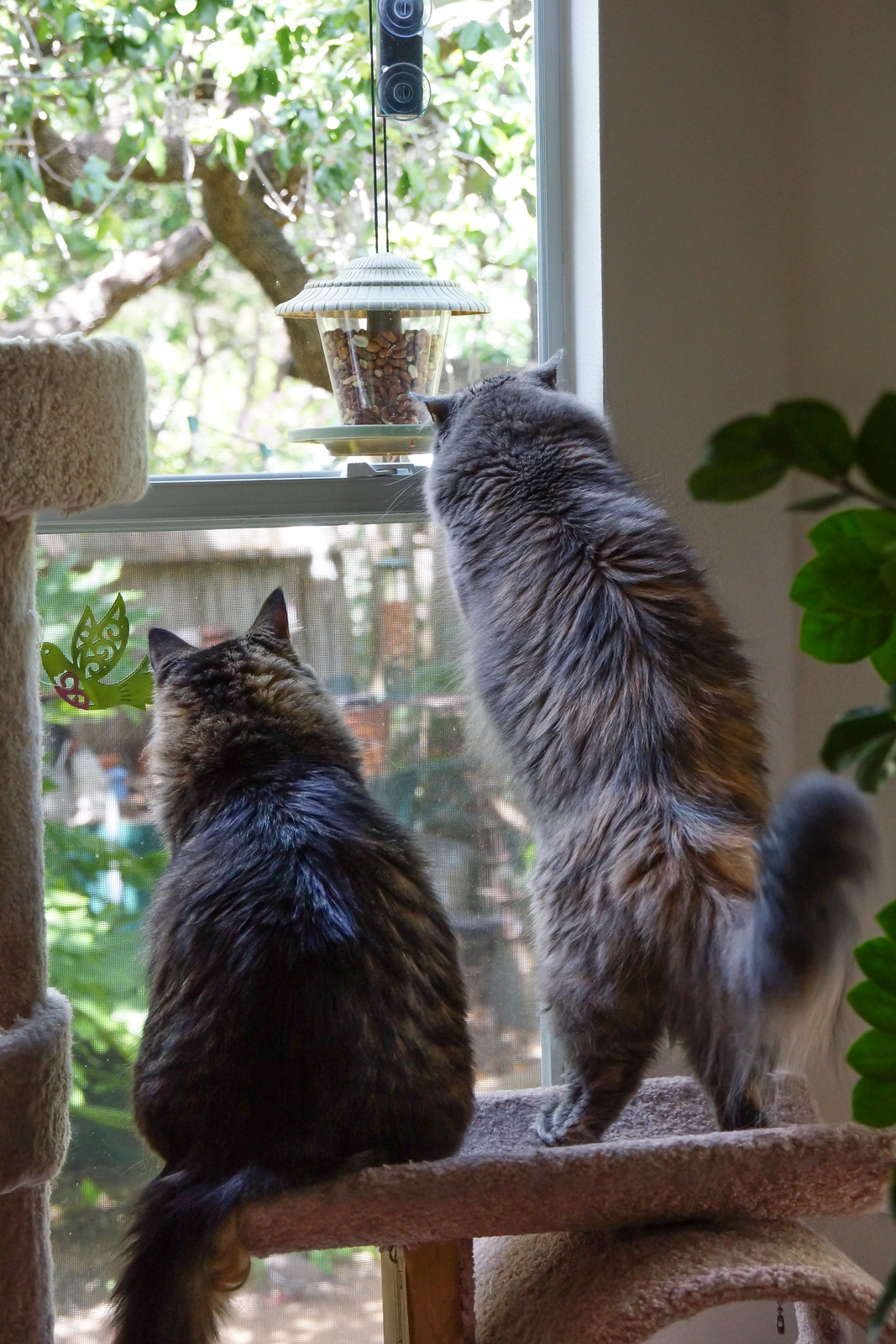In this detailed indoor photograph, we see two fluffy, long-haired cats intently gazing out through a large, bright window. The cats, one with a distinctive gray and orange fluffy tail and the other slightly darker, are perched on a short cat tower that doubles as a scratching pad. Next to them is an indoor potted plant, adding a touch of greenery to the scene. Directly outside the window, a bird feeder filled with pellets is visible, attracting the cats' attention. They appear captivated by the outdoor view of a backyard adorned with lush, green-leafed trees and various plants. A taller cat tower stands nearby, though the cats are not using it at the moment. The room's corner is subtly visible, featuring white walls and a chair with gray fabric, creating a cozy indoor setting from which the cats vigilantly survey the outside world.